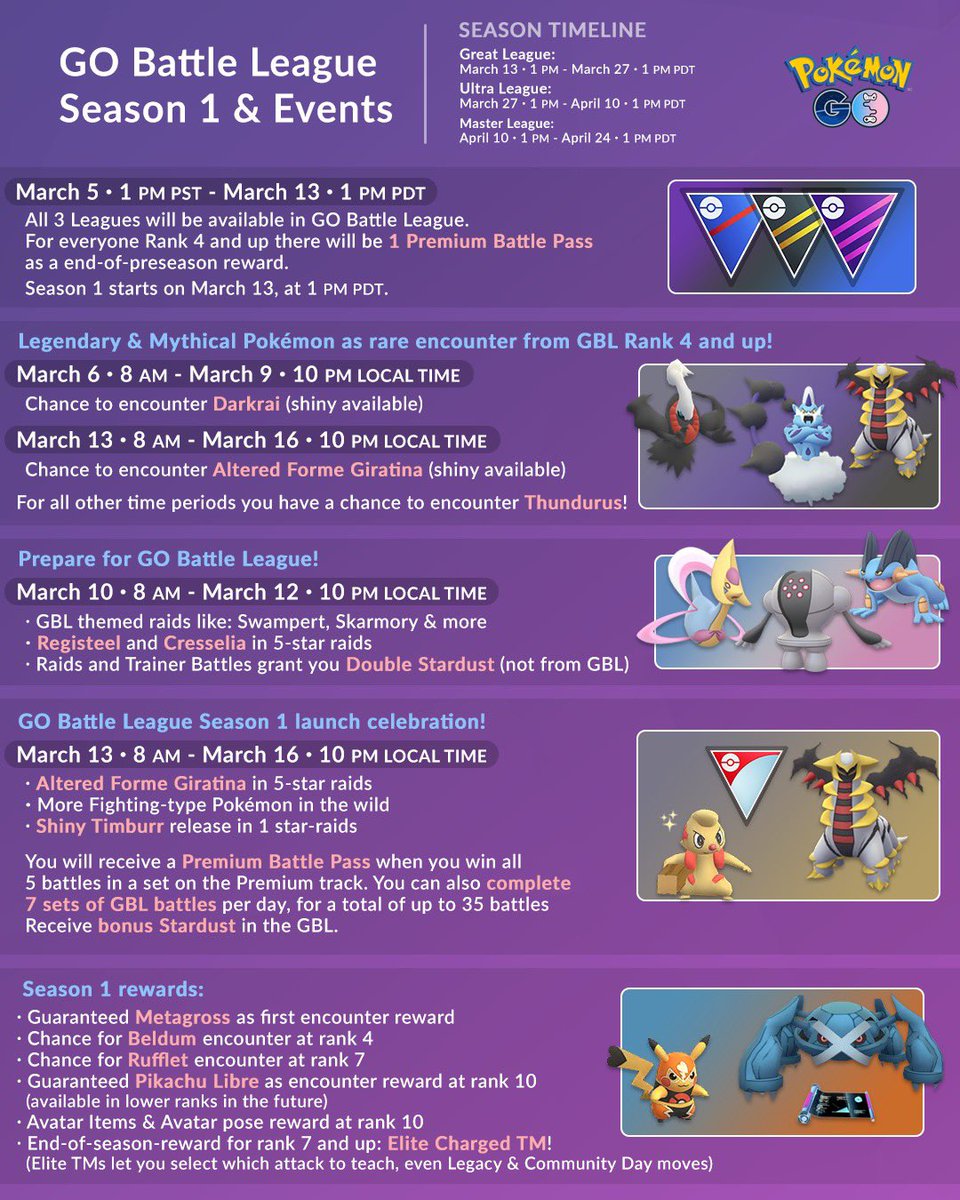This infographic screenshot features a brightly colored purple background with detailed white font text outlining the "Go Battle League Season 1 and Events". At the very top, the title "Go Battle League Season 1 and Events" is prominently displayed.

To the right of the title, a section labeled "Season Timeline" provides specific dates and times for the different league periods. The Great League runs from March 13th at 1 PM to March 27th at 1 PM PDT. The Ultra League follows, taking place from March 27th at 1 PM to April 10th at 1 PM PDT. Finally, the Master League is scheduled from April 10th at 1 PM to April 24th at 1 PM PDT.

An icon of the Pokémon symbol appears next to a Pokéball and the letter "G", symbolizing Go Battle League. Below this, there is a detailed list of events, rendered in white font. It specifies that on March 5th at 1 PM PST until March 13th at 1 PM PDT, all three leagues will be made available in the Go Battle League for participants of rank 4 and higher. Additionally, it mentions that a premium battle pass will be awarded as an end-of-preseason reward. The official start of Season 1 is noted to begin on March 13th at 1 PM PDT.

To the right of this text, there's an icon featuring three hanging banner flags, accompanied by the note: "Legendary and Mythical Pokémon is a rare encounter for trainers from Go Battle League rank 4 and up," occurring between March 6th at 8 AM and March 9th at 10 PM local time.